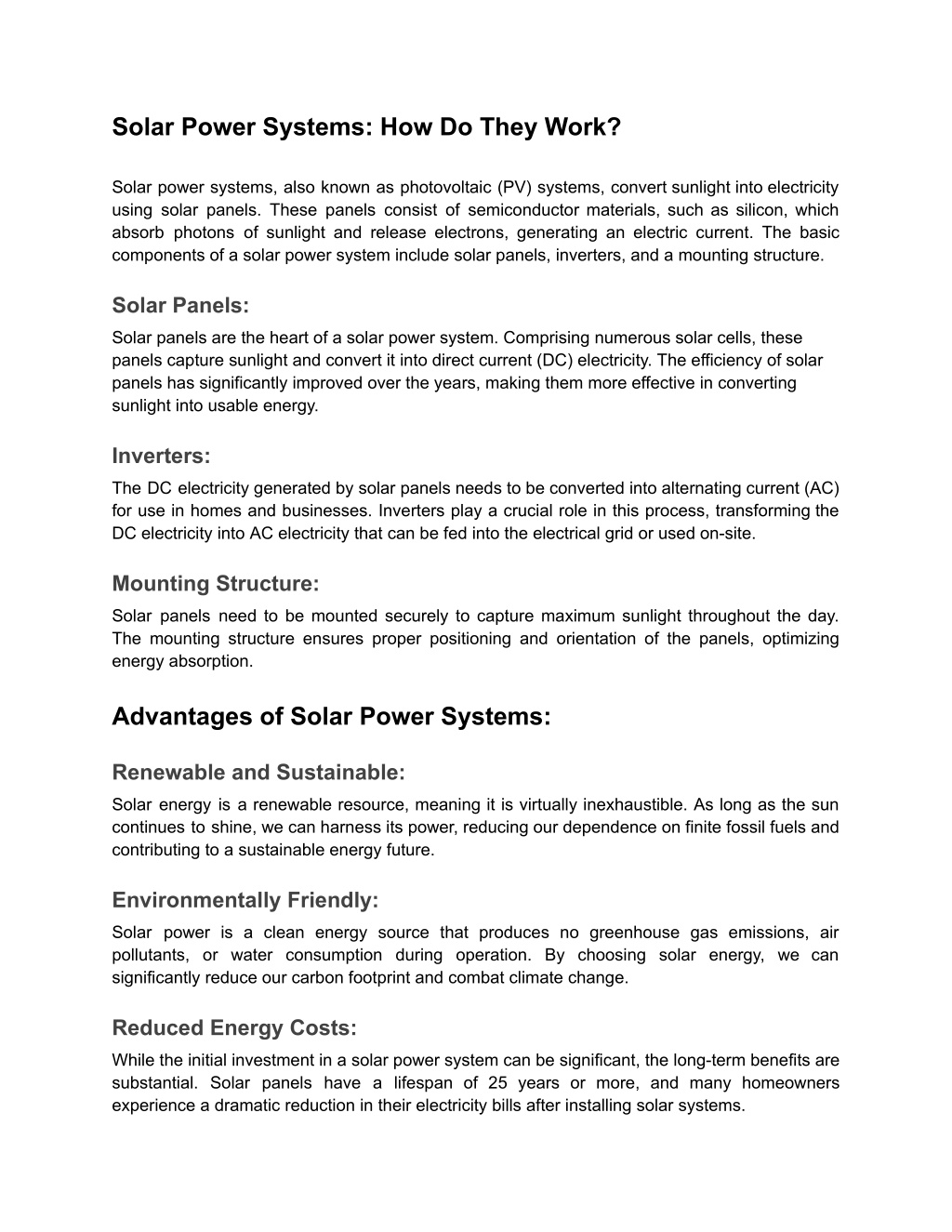This image displays a detailed article about solar power systems, comprising various sections and subcategories. The article begins with an introductory paragraph, offering an overview of photovoltaic (PV) systems and their role in capturing solar energy through solar panels.

The first main section is titled "Solar Power Systems: How Do They Work?" It breaks down the components and functionalities of a solar power system into three subcategories:
1. **Solar Panels** - A short paragraph explains how these panels capture sunlight and convert it into electricity.
2. **Inverters** - This paragraph describes the device's role in converting the DC electricity generated by the panels into AC electricity for home use.
3. **Mounting Structure** - The final paragraph in this section discusses the physical framework that supports the solar panels.

The second main section is "Advantages of Solar Power Systems." It elaborates on the benefits of transitioning to solar energy through three subcategories:
1. **Renewable and Sustainable** - This paragraph emphasizes the inexhaustible nature of solar energy.
2. **Environmentally Friendly** - This part highlights the ecological benefits, such as reduced carbon emissions.
3. **Reduced Energy Costs** - The final paragraph describes the financial savings associated with lower utility bills.

Each subcategory in both sections is concisely detailed in a single paragraph, making the image a comprehensive yet straightforward guide to understanding the framework and benefits of solar power systems.